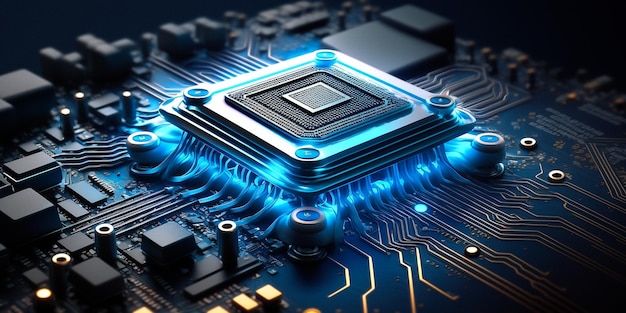This image depicts an intricate, digitally rendered computer chip set against a black circuit board background. At the core, a prominent CPU chip is centrally positioned, surrounded by a series of progressively larger squares, creating a sense of layered depth. The chip emits a striking blue neon light that accentuates its modern and high-tech appearance. The circuitry boasts intricate detail, with fine gold and black lines - resembling wires - branching out from the chip, connecting various components. Around the CPU, four circular elements, possibly representing screws or grommets, add to the structural complexity. The entire arrangement is viewed from an approximately 85-degree angle, emphasizing the three-dimensional, borderline fantastical nature of the design. The edges of the image blur into darkness, drawing focus to the brilliantly illuminated central chip, symbolizing its power and sophistication in a vividly futuristic and contemporary aesthetic.